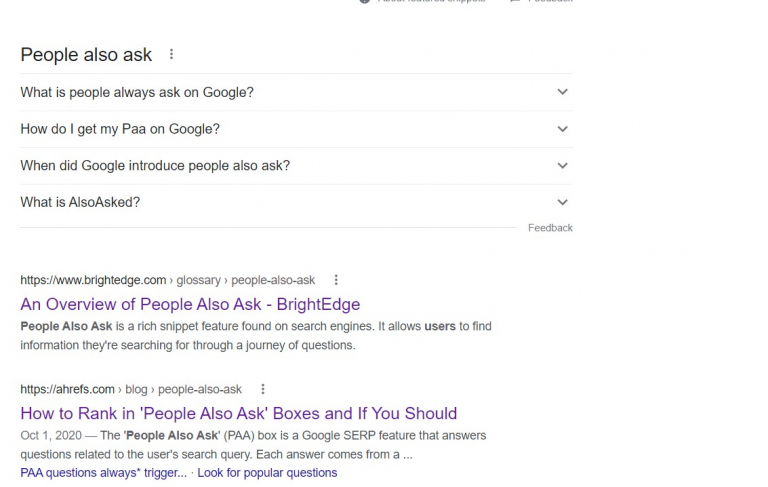A cropped image of a Google search results page likely viewed on a desktop. The top portion of the page, including the search bar and Google logo, is cut off, leaving only the bottom edges of text, which are entirely illegible. Despite this, the distinct Google layout is immediately recognizable. 

The visible section highlights the "People Also Ask" (PAA) panel, consisting of a white background with black text. Each entry in this panel features a downward-pointing arrow, indicating that a click would reveal additional information, though these details are not visible in the image. The questions listed in the PAA section are: 
1. "What is people always ask on Google?"
2. "How do I get my PAA on Google?"
3. "When did Google introduce people also ask?"
4. "What is also asked?"

Beneath the PAA panel, the typical Google search results layout is apparent, featuring URLs, clickable links, and descriptive blurbs. The two discernible results are:
1. "An overview of People Also Ask - BrightEdge," which describes the PAA feature as a rich snippet that helps users find information through a series of questions.
2. "How to rank in People Also Ask boxes and if you should," explaining that the PAA feature provides answers related to the user's search query.